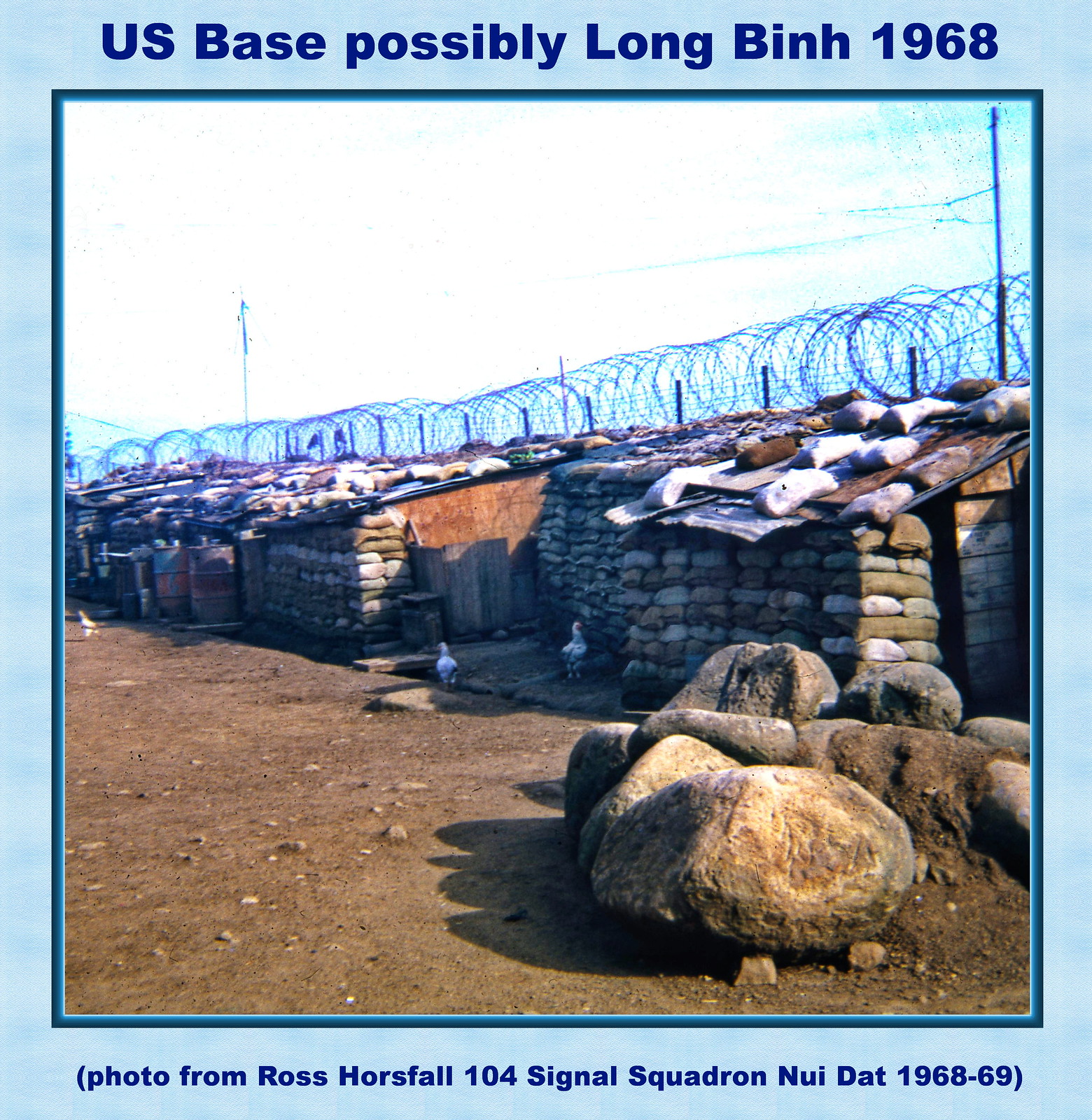The image, bordered in light blue, captures a moment from 1968 at a U.S. base, possibly Long Binh, in Vietnam. The top of the image features the dark blue text: "U.S. base, possibly Long Binh, 1968," while the bottom notes, "Photo from Ross Horsfall, 104 Signal Squadron, Nui Dat, 1968-69." The scene within depicts a dirt-filled ground with scattered boulders and makeshift shelter structures fortified with bags and rocks. Barbed wire coils form a protective fence around the area. A few white chickens roam the ground, adding life to the otherwise utilitarian military setup. The clear, bright blue sky casts distinct shadows, indicating a sunny day.